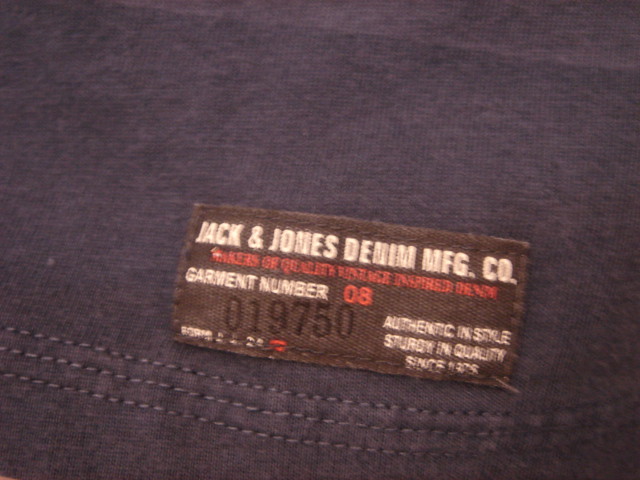The image features a close-up of a brownish-gray tag attached to a garment made of dark blue denim fabric, likely a pair of jeans. The tag, which appears somewhat blurry, reads in white print at the top "Jack and Jones Denim MFG. Co." Beneath that, in red text, it says "Makers of Quality Vintage Inspired Denim." Further down, it reads "Garments Number" in white, followed by "08" in red. Below that, there's a serial number "019750" in black. The tag also includes the phrase "Authentic in Style, Sturdy in Quality Since 1975" in white. The denim fabric, possibly a garment such as jeans or a denim shirt, displays visible stitching in three rows, emphasizing the quality craftsmanship. The color of the denim appears dark blue with a hint of purple, possibly due to the yellowish lighting in the image.